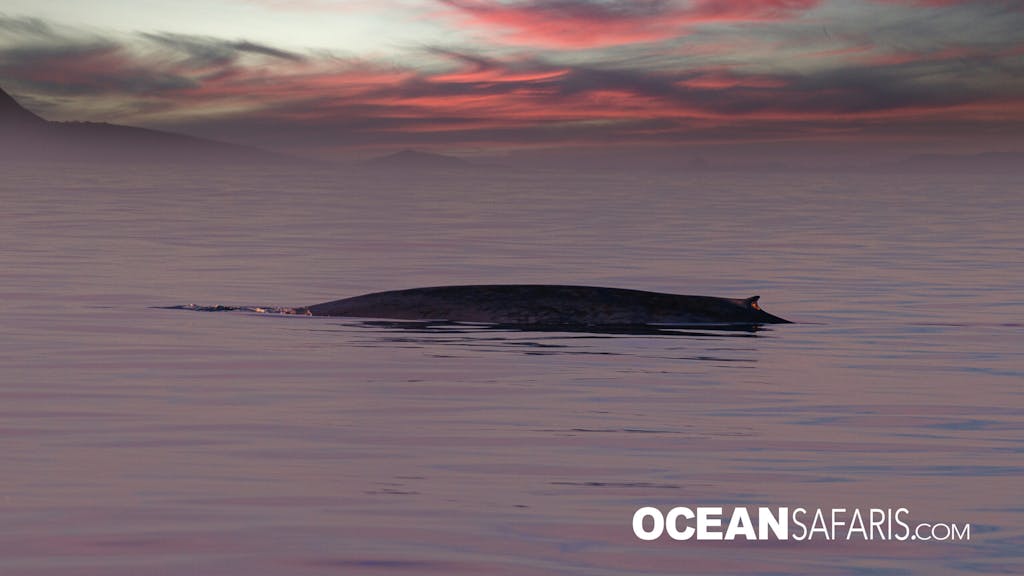This photograph by OceanSafaris.com, as indicated by the white watermark in the bottom right corner, captures a serene and enigmatic scene of the ocean at dusk. The still, reflective water occupies the majority of the frame, tinged with a stunning gradient of purple-pink hues that mirror the vivid sunset sky above. The sky itself is a dramatic blend of deep coral pink, red, and lavender gray, with patches of muted teal blue and lingering clouds that seamlessly fade into the horizon. Rising from the center of the image is the long, dark silhouette of a sea creature, likely the back of a whale, suggesting movement just below the water's surface with a visible blowhole towards one end. Subtle ripples around the breaching creature enhance the mystique, while distant mountain ranges are faintly discernible through the fog. This evocative image balances the tranquil beauty of the ocean with an underlying sense of mystery surrounding the creature.